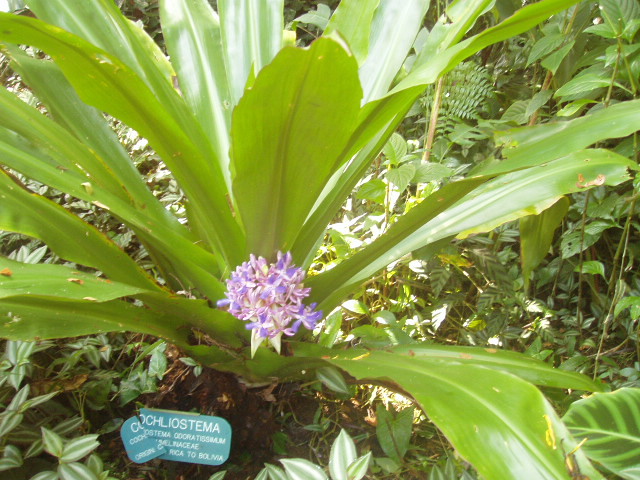This detailed caption describes a vibrant scene centered on a unique plant in an outdoor setting. The focal point is a plant with striking features—light purple flowers or a central bloom, accented with hints of white or yellow. Surrounding the bloom are large, light green leaves with prominent spines, some showing signs of yellowing or browning around the edges. The plant's leaves emerge radially from the ground, lacking a central stalk.

Nestled at the base of the plant is a torn blue sign, tilted slightly to the left, bearing the name "Cochliostema" in white letters alongside additional, smaller text that is mostly illegible. This sign seems to provide the scientific name or classification of the plant.

The scene is well-lit with bright sunlight casting a warm glow, which enhances the vivid colors of the foliage and accentuates the variegated greens. To the left and lower parts of the image, other plants with distinct features—such as striped leaves in silver and green—add to the diversity. Ferns and various green vegetation form a lush backdrop on the right and left sides, affirming the impression of a botanical garden or a similarly curated plant display area. The sunlight not only illuminates the main plant but also creates interesting shadows on the ground, further enriching the visual texture of the scene.